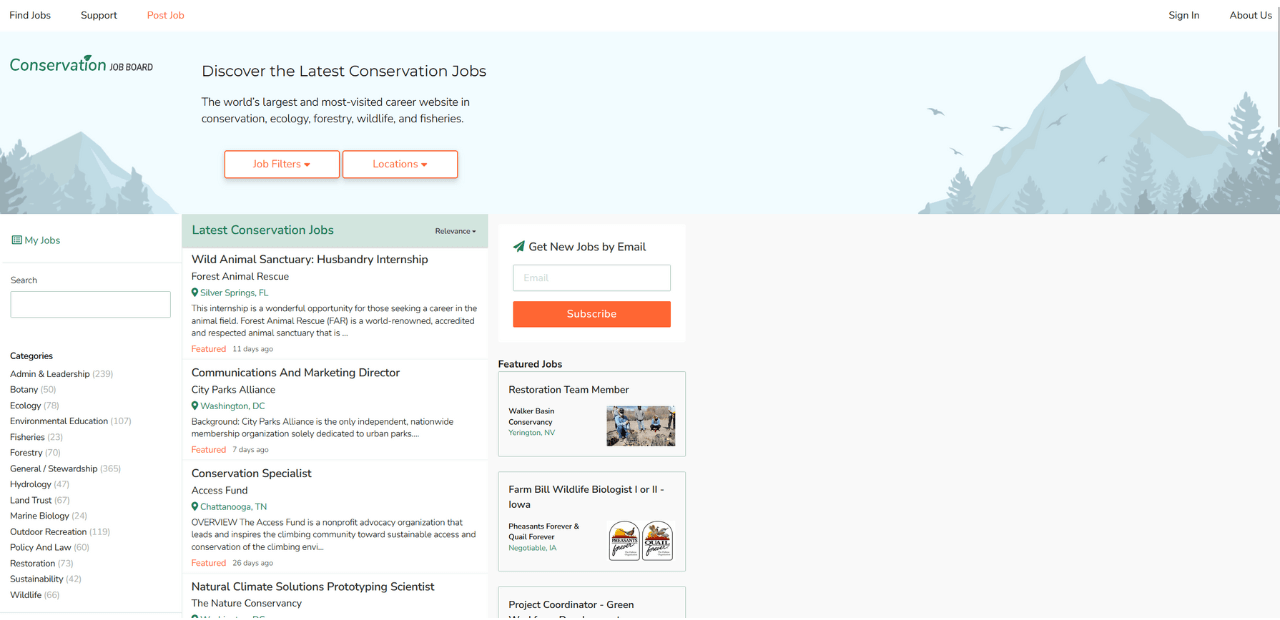The webpage depicted is a comprehensive conservation career platform, possibly the world's largest and most visited site for such opportunities. The user interface is divided into distinct sections aimed at job seekers in the conservation field.

Occupying the top third of the landscape-oriented screen, a picturesque banner showcases rugged mountains, majestic birds, lush trees, and an expansive sky, immediately communicating the site's focus on nature and environmental preservation. The header prominently features the word "Conservation," reinforcing the theme, and encourages users to "Discover the Latest Conservation Jobs."

The lower two-thirds of the screen split into two main sections: one half remains largely blank, while the other half is neatly organized into three vertical segments. 

- **First Segment: "My Jobs"**
  - This includes a search box for personalized job queries.
  - Below the search box are categories, presumably sorted for easy navigation through various conservation-related job types.

- **Second Segment: "Latest Conservation Jobs"**
  - This area highlights four recently posted job opportunities, offering a quick glimpse of available positions for users to explore.

- **Third Segment: "Get New Jobs by Email"**
  - A user-friendly subscription form invites visitors to input their email address to receive regular updates on new job listings, ensuring they stay informed about the latest opportunities in the conservation sector.

Filters and location drop-down menus at the top of the page facilitate refined searches, enhancing the user's ability to find relevant job openings efficiently. This structured layout clearly reflects the site's mission: connecting individuals with career opportunities dedicated to the preservation and protection of the natural world.